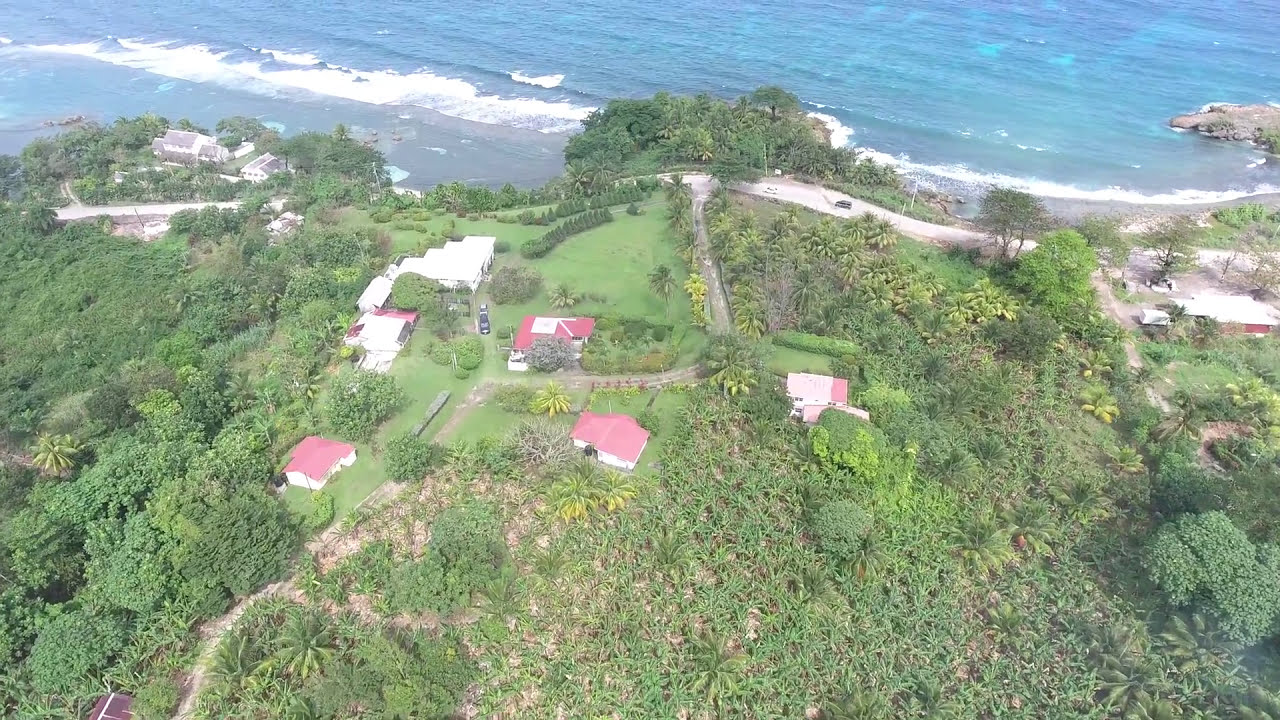The image is an aerial view of a lush, tropical beachfront community, likely taken from a drone high above the landscape. The foreground reveals a verdant, hilly area densely covered with dark green trees, including palm trees, interspersed with neatly clipped grass and occasional patches of weeds. Several buildings are scattered across the scene, showcasing a mix of structures with red roofs and white walls, along with some distinctive buildings such as a white-roofed house and another with a gray, arched roof positioned in the far left corner.

A winding, twisty street meanders through this neighborhood, further enhancing its picturesque appearance. Beyond the greenery, the scene opens up to a stunning coastline. The ocean water is a mesmerizing blend of bright blue and light green-teal hues, with visible coral formations beneath its surface. White waves froth as they approach the sandy beach, creating a vivid contrast against the shoreline. The entire setting evokes a serene, tropical paradise, reminiscent of locations like Hawaii, though the altitude of the shot prevents the identification of any individuals on the beach below.